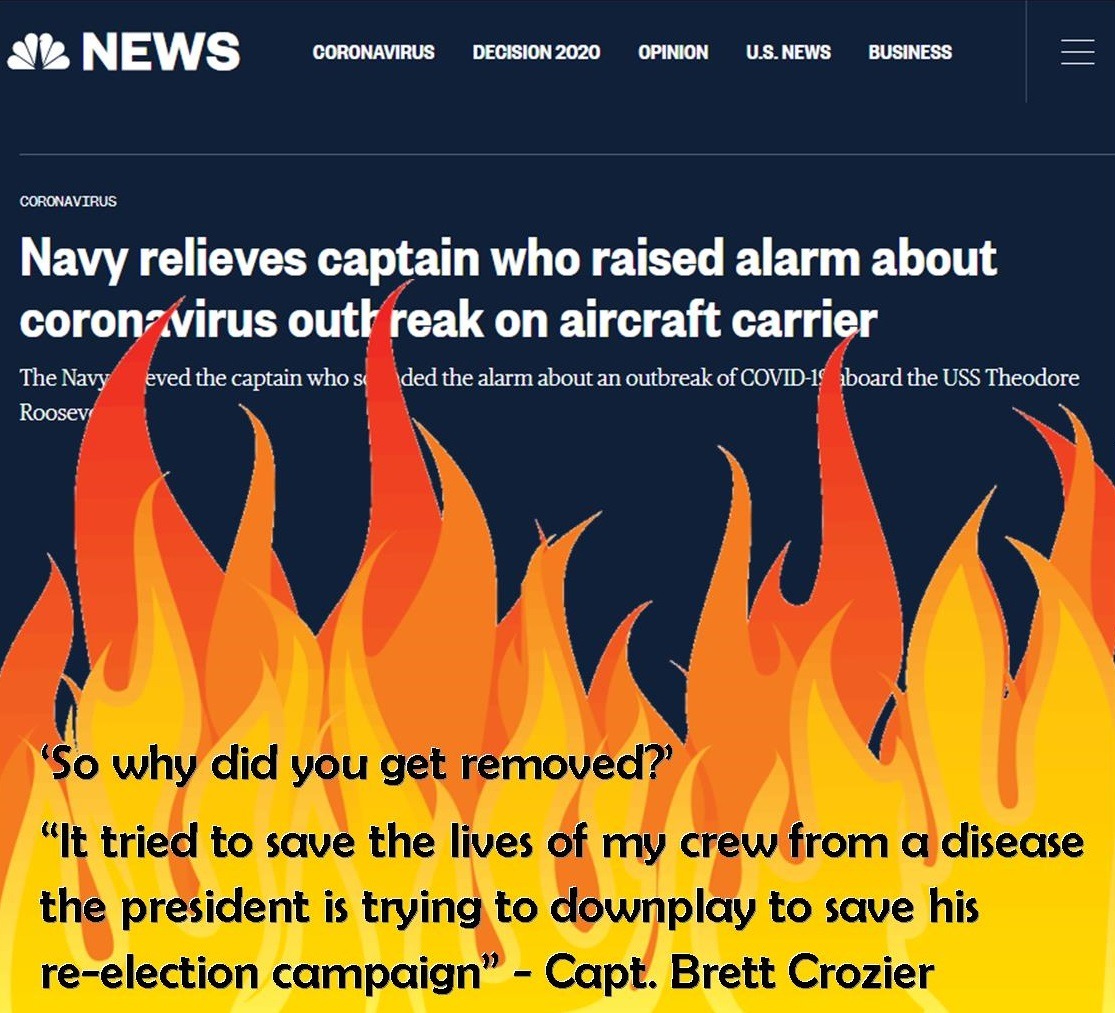In this screenshot, we observe a section of a web page. The upper left corner of the page features a black background with an illustration of flames rising from the bottom. At the top, the title "News" is displayed, accompanied by the NBC iconic logo to the left. Below the title, a series of categories are listed in white text: "Coronavirus," "Decision 2020," "Opinion," "US News," and "Business." 

A thin, horizontal gray line separates these elements from the main content below. Under the gray line, "Coronavirus" is written in small white text. Below it, a bold, larger white text headline reads: "Navy Reliefs Captain who raised alarm about Coronavirus outbreak on aircraft carrier."
 
Within the flames' illustration, there is a highlighted quote: "So why did you get removed? I tried to save the lives of my crew from a disease the President is trying to downplay to save his re-election campaign," attributed to Captain Brett Crozier.